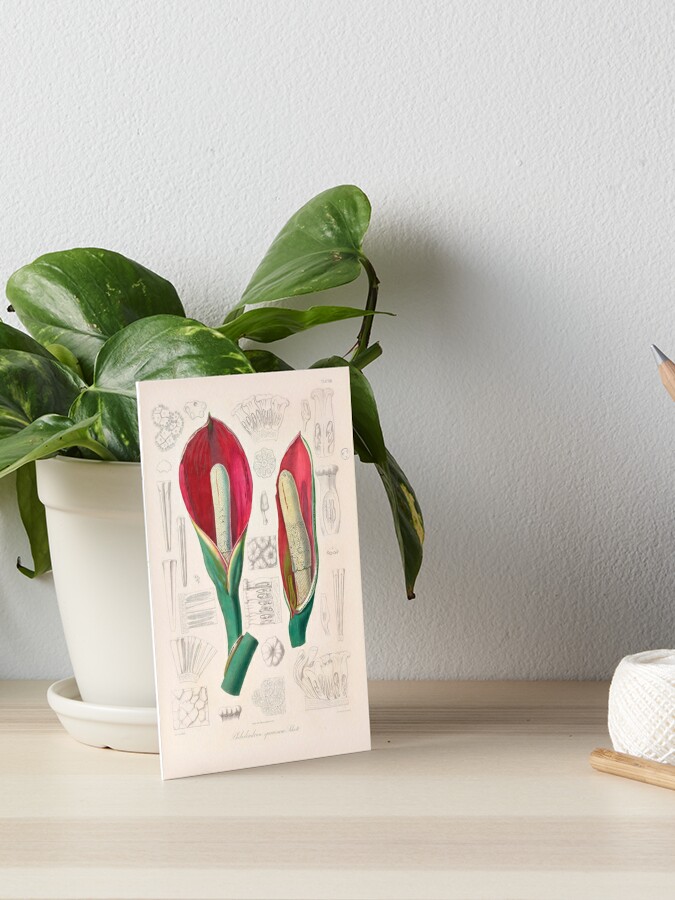The image showcases a small, vibrant green plant with heart-shaped leaves, housed in a sleek white ceramic or plastic pot with a matching saucer. The plant appears healthy, with several medium-green leaves extending upwards and some gracefully hanging over the side. The setting includes a light, blonde wooden shelf against a grayish-toned wall, offering a minimalist backdrop. 

In front of the plant is a greeting card displaying artistic illustrations of calla lily blossoms. The flowers on the card feature red petals with elongated white stamens in the center, emerging from green stems. The card also contains various diagrams and black markings, adding a detailed element to the scene. To the right of the setup lies a roll of twine, subtly contributing to the natural aesthetic.